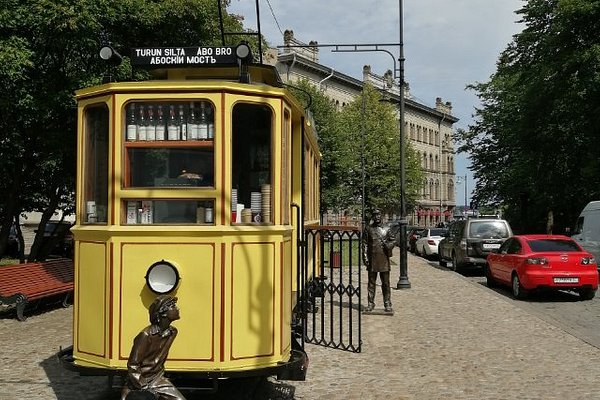In a bustling urban setting, likely somewhere in Europe, the focal point of this outdoor scene is a stationary yellow trolley car adorned with red stripes. This vintage vehicle, reminiscent of a streetcar or food truck, features a striking black sign with white text reading "Turin, Silta, ABBRO," alongside additional letters that are difficult to decipher. The trolley appears to be a unique vendor, showcasing wine bottles on the top shelf and cups on a counter below, suggesting it serves drinks. Encircling the trolley are several small bronze statues, including one directly in front of it and another to its right.

The scene extends to include a tree-lined street where a few cars, including a red sedan, a black Jeep, and a white car, are parked or possibly in motion. Adjacent to this street, there's a black streetlight pole and a park bench situated on a cobblestone or beige stone sidewalk. Further in the background, a formidable four-story stone building with a rectangular facade stands against the backdrop of a clear blue sky. Altogether, this meticulously detailed scene captures the vibrancy and charm of a European urban landscape.